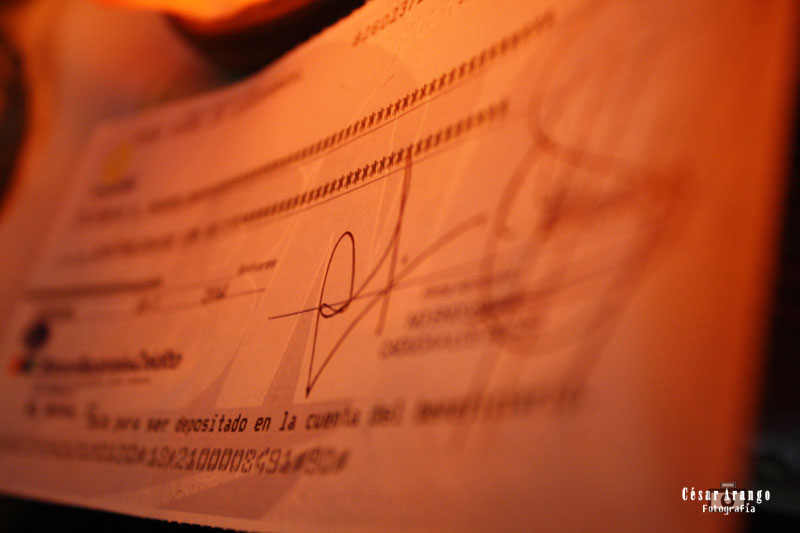This image features an extreme close-up of a commercial-sized check, likely from a Spanish-speaking country, captured under low light conditions that lend an orange and black tint to the scene. The close-up reveals intricate details of the check, including what appears to be a series of micro-numbers at the bottom, resembling routing and account numbers typically found on bank checks. The focal point of the image is a signature, which looks like two initials with a distinct, elaborate flourish. Although much of the text surrounding these elements is blurry and hard to decipher, you can make out Spanish words such as 'Seattle,' 'Ian,' and 'Corella.' The check also features rows of small, cut-out figures as part of its design. In the bottom right corner, the words "Cesar Arango Fotografia" are visible, accompanied by a small camera icon, indicating the photographer's watermark.